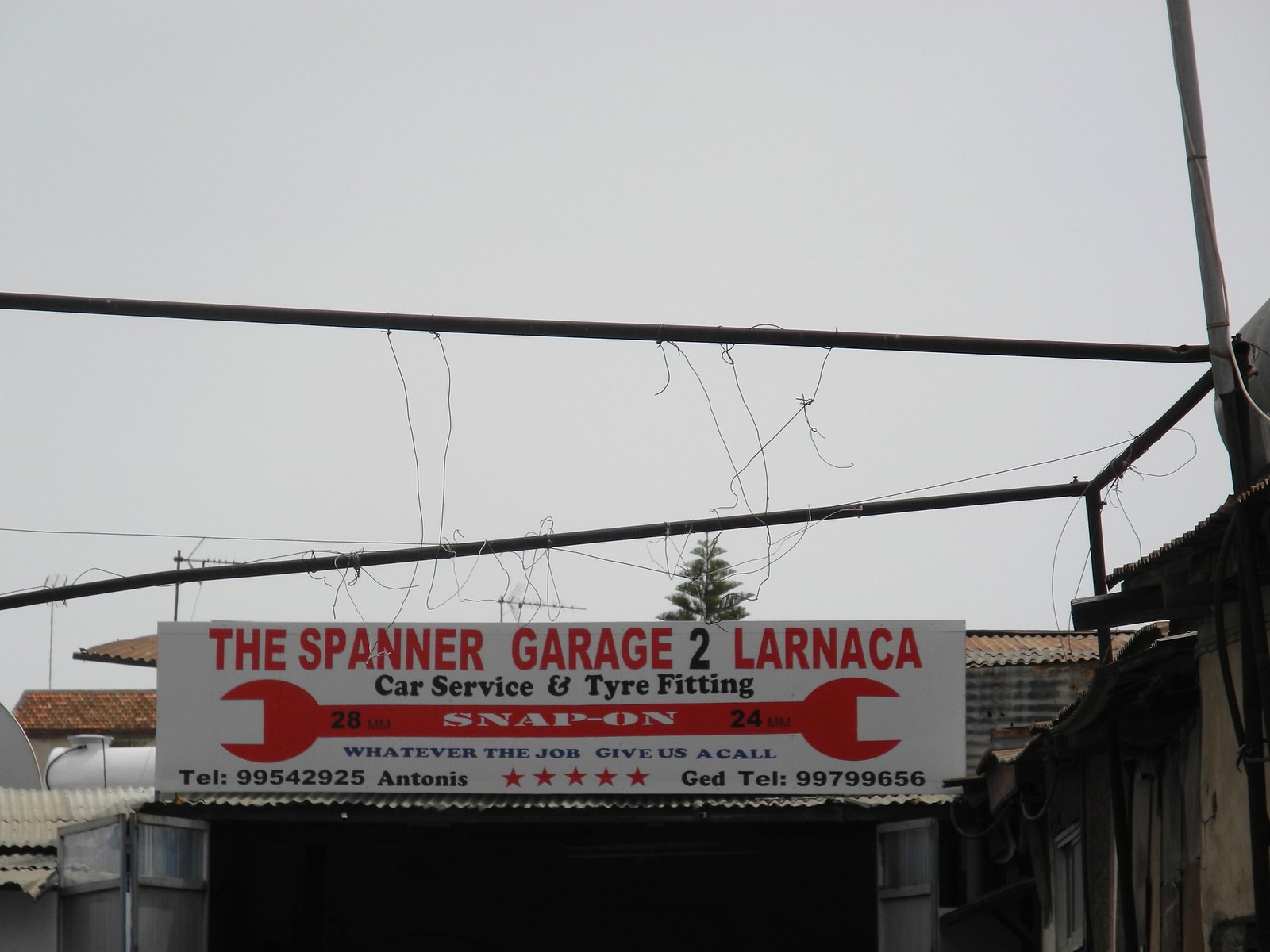The photograph depicts the front of a garage building under a gray sky, characterized by its corrugated metal walls and roof. Above the garage door is a prominent white sign with a long, skinny shape. The top portion of the sign features bold red capital letters spelling "THE SPANNER GARAGE 2 LARNACA." Below, in smaller black text, it reads "Car Service and Tire Fitting," with "Tire" notably spelled with a "Y." Spanning the width of the sign is an image of a red double-headed wrench, marked with "SNAP-ON" in the center in white font. One end of the wrench displays "28mm" and the other end "24mm." Beneath the wrench, in black text, it says "Whatever the job, give us a call," followed by two phone numbers and a row of five stars in between. The structure is surrounded by various metal poles and bars, and there is a tree visible in the background. To the side, another building can be seen partially within the frame.